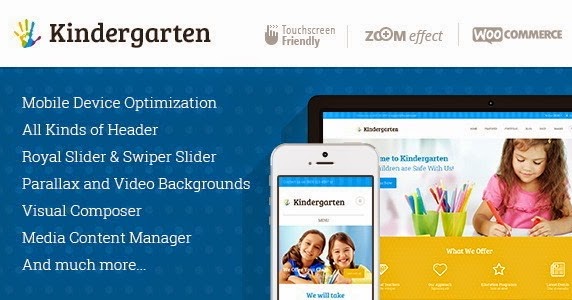The image features a vibrant, educational-themed layout designed to highlight an interactive, user-friendly kindergarten platform optimized for various devices. In the top left corner, the word "Kindergarten" is prominently displayed in bold, black lettering accompanied by a colorful handprint logo to its left, adding a playful touch. The background of the image is a soothing blue, which creates a pleasant contrast to the white text scattered throughout the layout.

Key features outlined across the image include "touchscreen friendly" design, "zoom effect" capabilities, "WooCommerce" integration for e-commerce solutions, and "mobile device optimization" ensuring seamless access across smartphones and tablets. The image also emphasizes versatility with "all kinds of header" options, and advanced media presentation tools like "royal slider and swiper slider," alongside engaging "parallax and video backgrounds."

The detailed description extends to include tools for content creation and management such as "visual composer" and "media content manager."

The visual elements of the image consist of a photo of a cell phone screen displaying two children interacting on the device, symbolizing the app's accessibility and kid-friendly design. Additionally, there is an image of a laptop screen showing a young child next to coloring crayons and other art supplies, underscoring the app's creative learning aspect. This image effectively communicates a comprehensive, optimized, and engaging platform ideal for early childhood education.